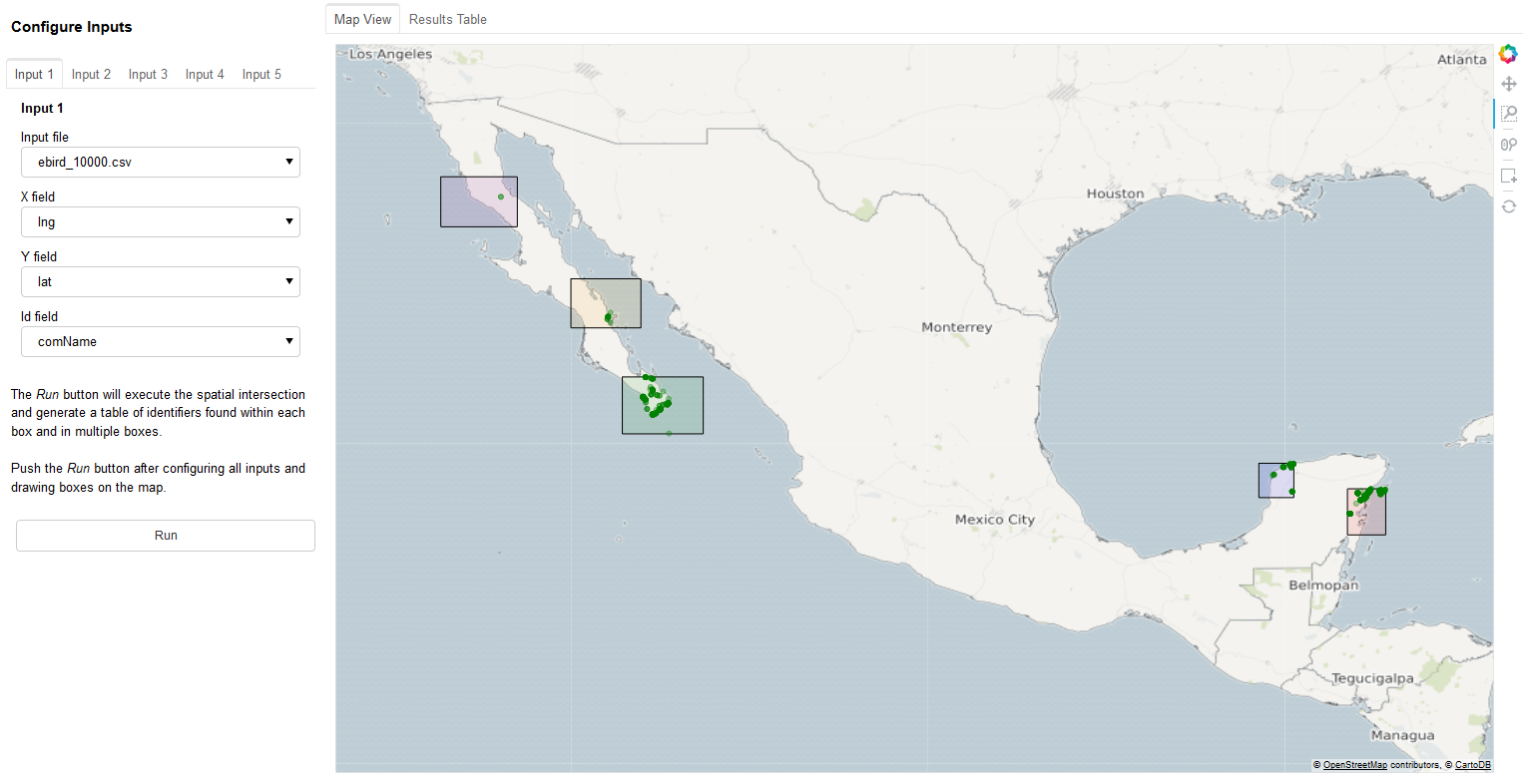This image features a detailed interface for configuring spatial data inputs and generating geospatial analyses, with a primary focus on a map occupying the majority of the right side of the page. 

To the left, there is a title at the top that reads "Configure Inputs," accompanied by five tabs labeled "Input 1," "Input 2," "Input 3," "Input 4," and "Input 5." "Input 1" is currently active. 

Beneath these tabs, the interface provides several input fields:
- **Input File**: Displays a specific file name.
- **X Field**: Includes a drop-down box with "LNG" selected.
- **Y Field**: Includes another drop-down box with "LAT" selected.
- **ID Field**: Features a drop-down box with "com name" selected.

A "Run" button is prominently displayed below these configurations, accompanied by explanatory text that outlines its function: executing a spatial intersection to generate a table of identifiers found within each drawn box and across multiple boxes on the map.

The map itself predominantly showcases Mexico, extending to include parts of the southern United States. Various cities are marked on the map, including:
- In the United States: 
  - Los Angeles (upper left corner)
  - Houston (center)
  - Atlanta (upper right corner)

- In Mexico:
  - Monterrey
  - Mexico City

Additionally, Central American cities such as Belmopan, Tegucigalpa, and Managua are labeled as well.

Several rectangular shapes are drawn on the map, enclosing specific regions that contain green dots, likely representing particular data points or locations of interest for the analysis.